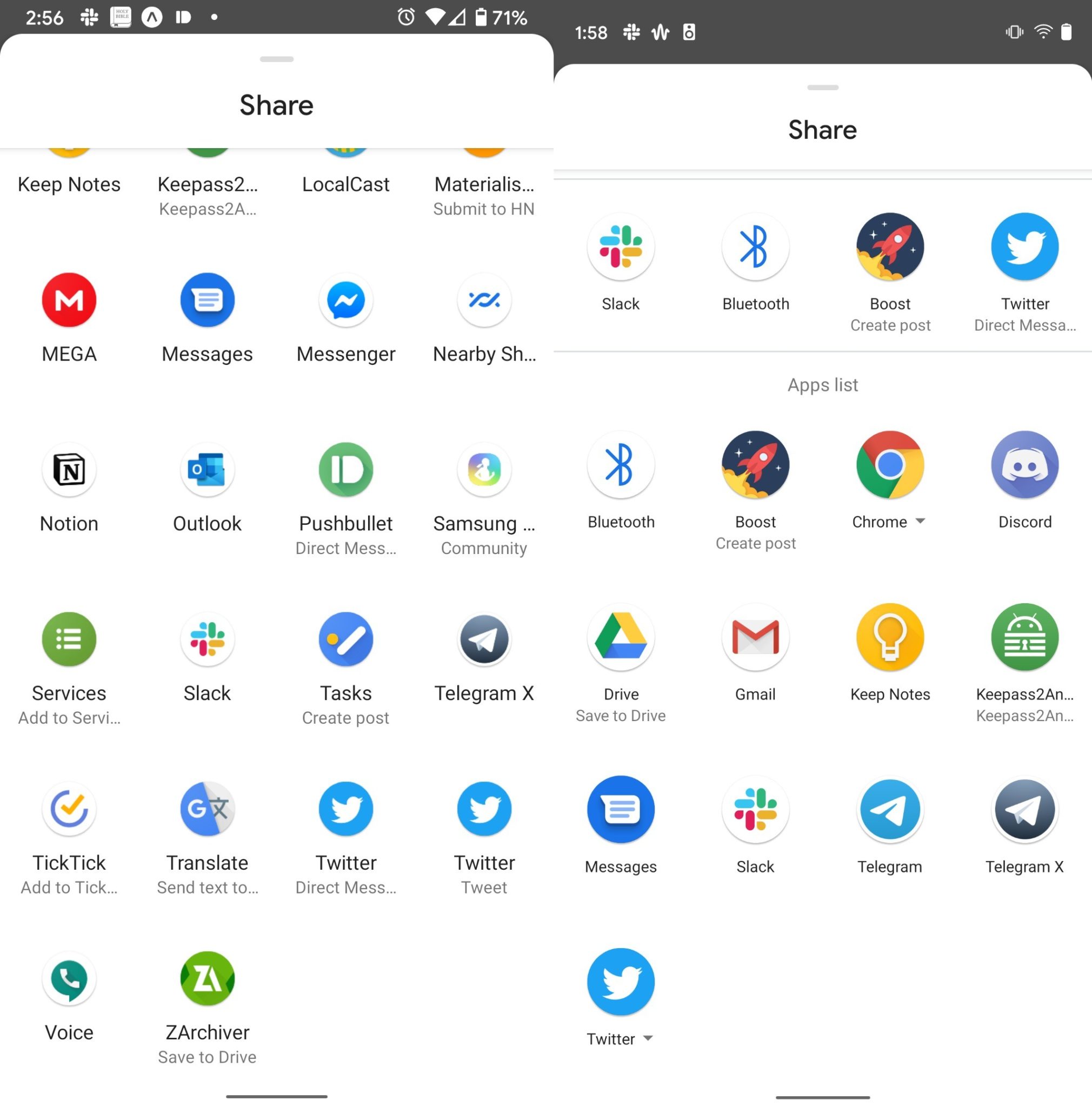Two screenshots display the "Share" menu of an Android phone. Both images showcase a grid of app icons on a plain, white background, which might initially resemble an app drawer but is actually the interface for sharing content. 

In the left screenshot, apps like Mega, Notion, Outlook, Pushbullet, and Twitter are visible. The right screenshot, though similar, includes different apps such as Boost, Chrome, Discord, Slack, Telegram, and also Twitter. Icons are uniformly presented within circular boundaries, and the word "Share" is prominently positioned at the top of each image. The primary difference between the two screenshots lies in the specific apps shown. While some apps overlap, others are unique to each image, demonstrating a diverse array of sharing options.